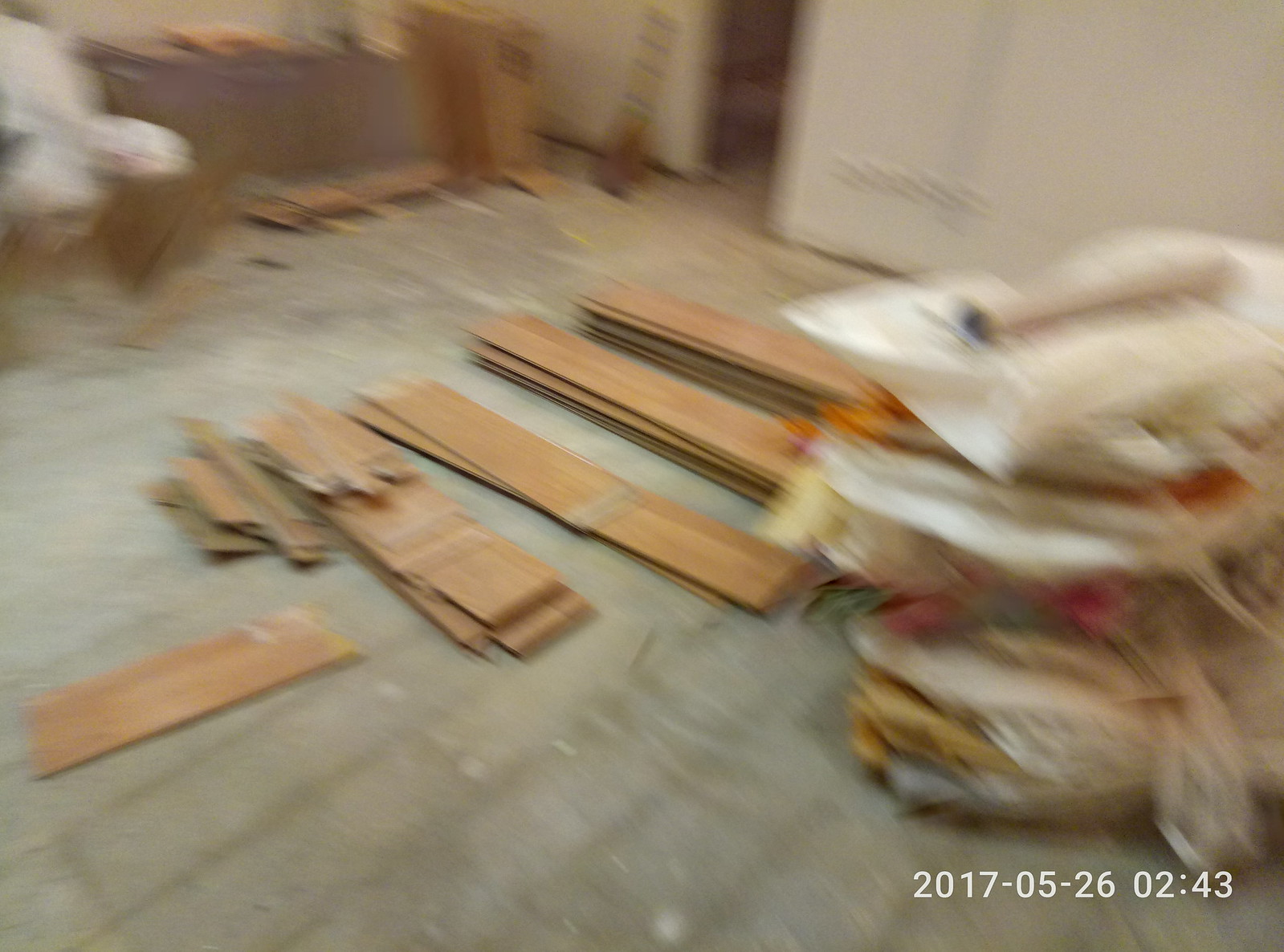In this slightly blurred colour photograph with a timestamp in the bottom right-hand corner reading "02:43" and a datestamp "2017-05-26," we observe a renovation project. The scene features a dusty cement floor with remnants of laminate flooring that has been torn up, leaving behind scattered planks, some broken and others splintered, stacked haphazardly. Evidence of previous moisture or staining is visible on the concrete where the laminate used to lie. The right foreground of the image contains a pile of white items that appear to be plastic bags, cloths, or packing materials. In the background, vague outlines of additional construction materials and possibly pieces of furniture or debris are visible, pushed to the side to facilitate the removal of the old flooring. The far-left corner shows something purple accompanied by another white object. Overall, the room is cluttered and disorderly, filled with various materials in different states of disarray, indicative of an ongoing renovation process.